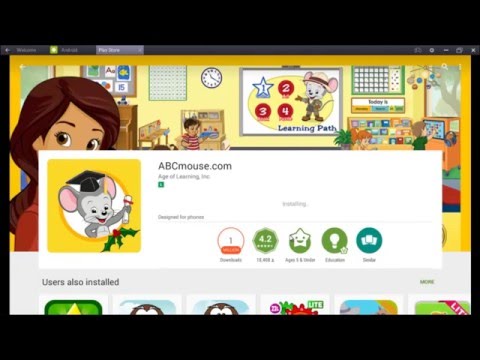The screenshot depicts a children's educational website, likely an app store page for a learning application. The screen is framed by black bars at the top and bottom. The main content area showcases a colorful, cartoon-style illustration of a woman in a classroom with children engaged in various activities. The classroom setting includes a board with a mouse and the text "Learning Path."

There's a prominent white overlay featuring a square image of a cartoon mouse wearing a graduation cap and holding a diploma. It includes text indicating "abcmouse.com, Age of Learning, Inc.," accompanied by approval icons related to educational quality and ratings, although the specific details are too small to read clearly.

In the lower part of the screen, there are indications of six game icons, partially visible and cut off. This suggests the user is navigating an app store, possibly the Play Store, and considering downloading this educational app. Due to the small font size and blurriness, additional text details are unreadable, but the overall context points to an app designed for children's learning.